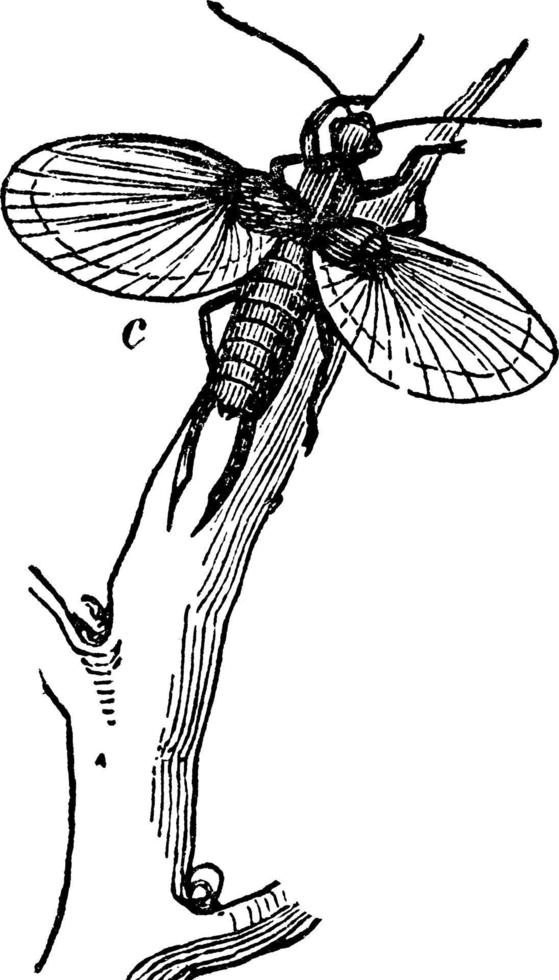The image showcases a detailed, black-and-white illustration of an insect perched on a simple tree branch, rendered in hand-drawn black pen ink. The insect, likely a type of fly, is depicted with two horizontally spread wings, two long antennas pointing upwards, and four legs positioned below it. Additionally, the insect features two talons protruding from its rear end. The branch, elegantly drawn with short offshoots, spans the scene with minimal shading along its right side and on the insect's body. The illustration is mostly composed of outlines without any color fill, leaving the unfilled spaces white, matching the background. A notable detail is the single letter "C" located underneath the left wing of the insect. The insect sits prominently towards the upper center of the image, lending a simple yet captivating focus to the drawing.